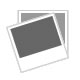This vertical rectangular image is somewhat blurry and glary, complicating the visibility of its details. Dominating the center, and extending from mid-right down diagonally and back up, is a white border that likely belongs to the top of a trash can or a bucket. Below this border, there are segments of orange, yellow, and brown. The glare seems to originate from two light gray lines descending from the top left to the bottom edge of the image, alongside a broader, lighter gray line to their right that also extends down and left before exiting the frame. Overlaid on this white-bordered object is a label with partially discernible writing; letters such as "E," "A," and a sequence "N D O L" can be seen on a light yellow surface, partly illuminated by the glare.

The image also features fine stripes or lines, possibly from a light source, adding to the glare effect. Although the object in question initially appears to be a cup, perhaps reminiscent of a Starbucks cup or a vintage Gibson or Stella cup, further examination reveals that it is actually a stringed instrument, specifically a guitar. The photo appears to be taken through its strings and sound hole, aiming to capture the label inside, which reads "N-D-O-L-I-N."

Additionally, the perspective suggests a view overlooking a cup-like structure, with contents resembling a candy, possibly a rolled-up chocolate wrapped in gold packaging. The image thus presents a complex interplay of light, reflection, and partial visibility, framed by the elements of the guitar and light interference.